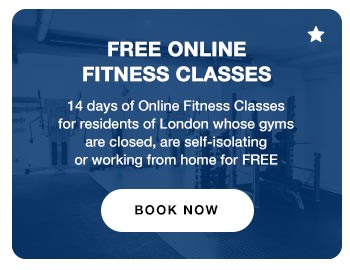This screen capture features a photograph of a gym, visible through a blue-colored tint that lends a somewhat murky quality to the image. In the background, one can observe various exercise machines, including weight lifting and resistance training equipment. Overlaid on this backdrop, text announces "Free Online Fitness Classes." It promotes a special offer providing fourteen days of complimentary online fitness sessions available to London residents who are affected by gym closures, self-isolation, or remote work requirements. The top right corner of the screen capture is adorned with a star, while a lozenge-shaped white button displaying the words "Book Now" in black is prominently positioned, inviting immediate action.